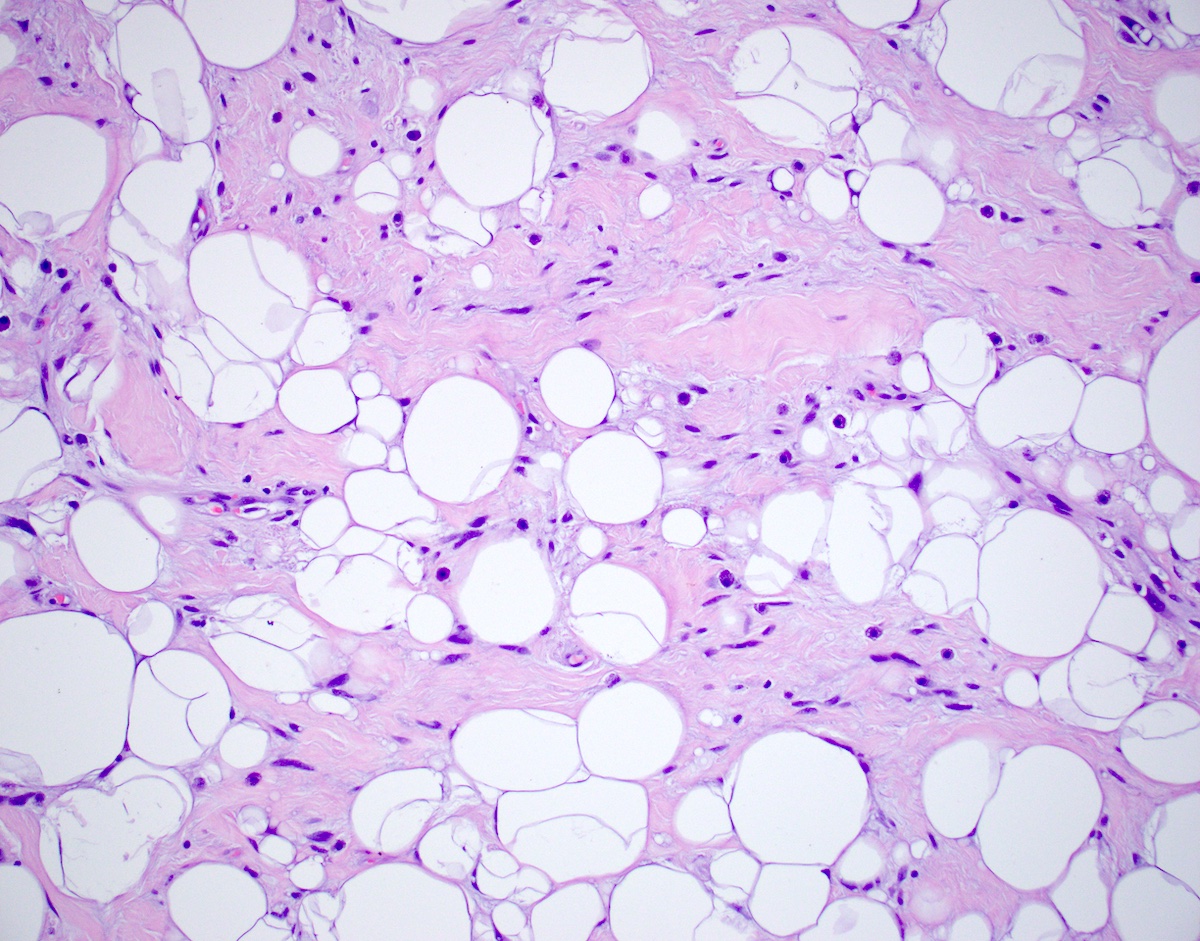This image appears to be a detailed microscopic view of a biological system, potentially cells or muscle tissue. The primary visuals include numerous white, circular shapes resembling bubbles, varying in size, and densely packed across the entire image. The background is a vibrant combination of light lavender and pink hues. Between the white circles, there is a flowing pinkish liquid interspersed with purple streaks, creating a dynamic and intricate backdrop. The white circles sometimes show faint lines across them, adding texture. The purple elements are scattered throughout, enhancing the complexity of the scene. Despite its scientific appearance, the arrangement and coloring suggest it could also be interpreted as an abstract piece of artwork.